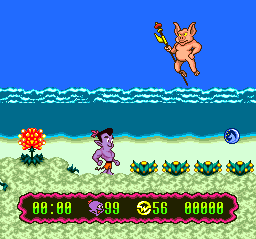This screenshot, captured from a video game, is a perfect square in shape. The bottom half of the image showcases various in-game statistics, highlighted by a red squiggly outline. These stats are prominently displayed in bright neon green numbers and letters against a black background, providing information on the player's performance in the game.

The top half of the screenshot depicts a vibrant in-game world featuring a beach scene. The sky is a brilliant blue, adding a sense of realism and depth to the environment. Flying in this bright blue sky is a pinkish-tan pig with elongated ears, gripping a blue pole with a red tip.

Below the flying pig, the beach is depicted with elements like water, grass, sand, and some flowers. In the center of this beachy landscape stands a purple-skinned character. This character sports dark black hair, red shorts, and a matching red hat, contributing to the colorful and whimsical nature of the scene.